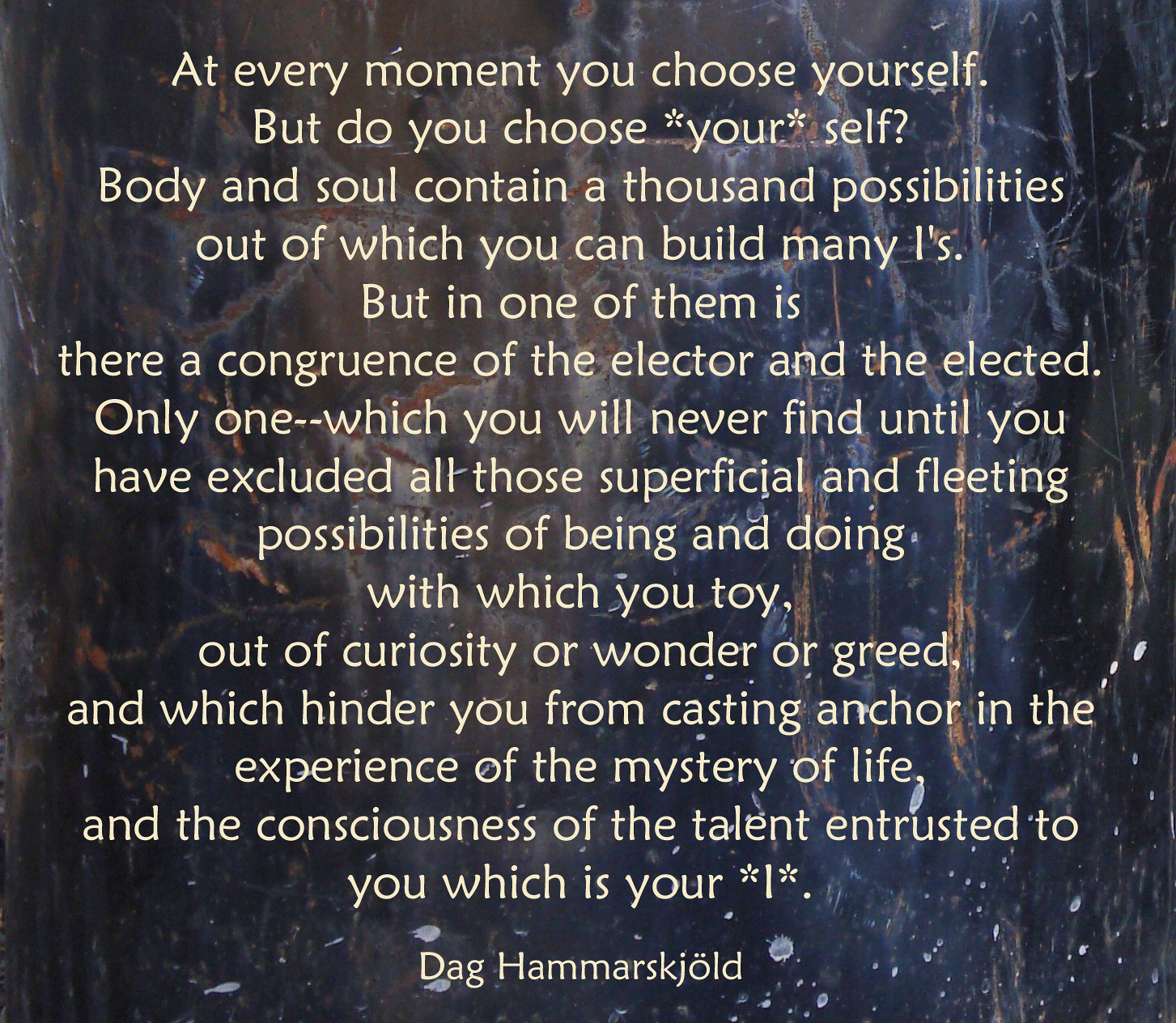The image is slightly longer than it is tall and showcases a passage by Dag Hammarskjold. The text, presented in light yellow, begins at the top and flows downward in an indented format. The background is an abstract composition with black as the dominant color, accented by splatters and streaks of orange, light blue, gray, and white dots, creating a dynamic and vibrant backdrop. The passage reads: "At every moment you choose yourself. But do you choose your *self*? Body and soul contain a thousand possibilities out of which you may build many *I*s. But in one of them is a congruence of the elector and the elected. Only one—which you will never find until you have excluded all those superficial and fleeting possibilities of being and doing with which you toy out of curiosity or wonder or greed, and which hinder you from casting anchor in the experience of the mystery of life and the consciousness of the talent entrusted to you, which is your *I*." The text concludes with the signature of Dag Hammarskjold, written with an "ö" in the last name.